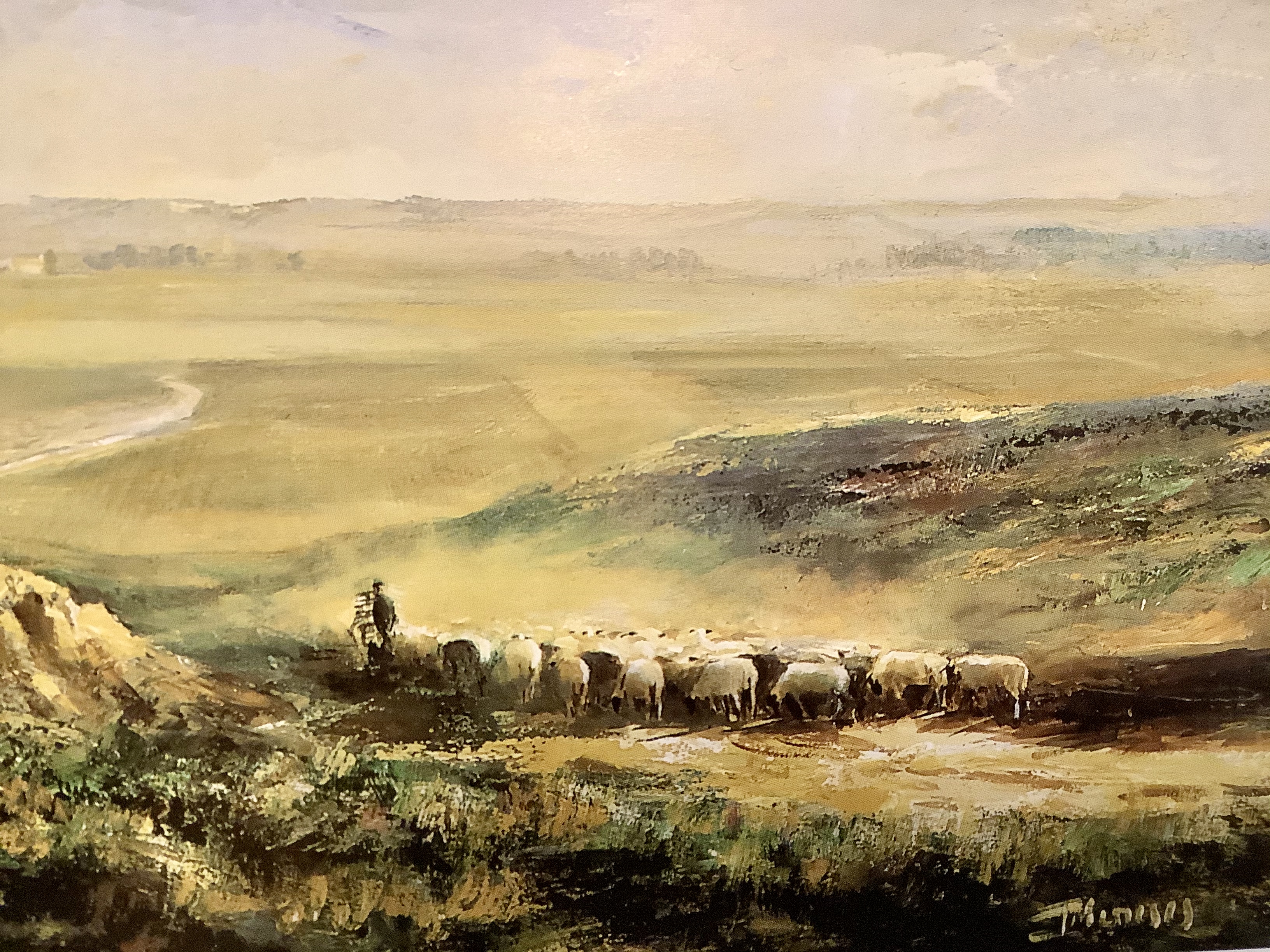This is a photograph of an oil painting that depicts a sheep herder guiding a flock of sheep across a vast, open field. The scene features rolling hills and grasslands in the background under a hazy sky with grayish-white clouds. The painting employs thick, somewhat abstract brushstrokes, contributing to its muted, earthy color palette of tans, browns, greens, and touches of blue. In the foreground, the sheep, primarily white with black faces, are grazing or being herded, moving away from the observer. The sheep herder, whose gender is indeterminate, is positioned on the left side of the image. The painting is signed in the bottom right corner with an illegible signature that appears to begin with the letter "T." Despite its abstract style, the pastoral scene is clear and evocative, capturing the tranquil yet dynamic movement of the herd.